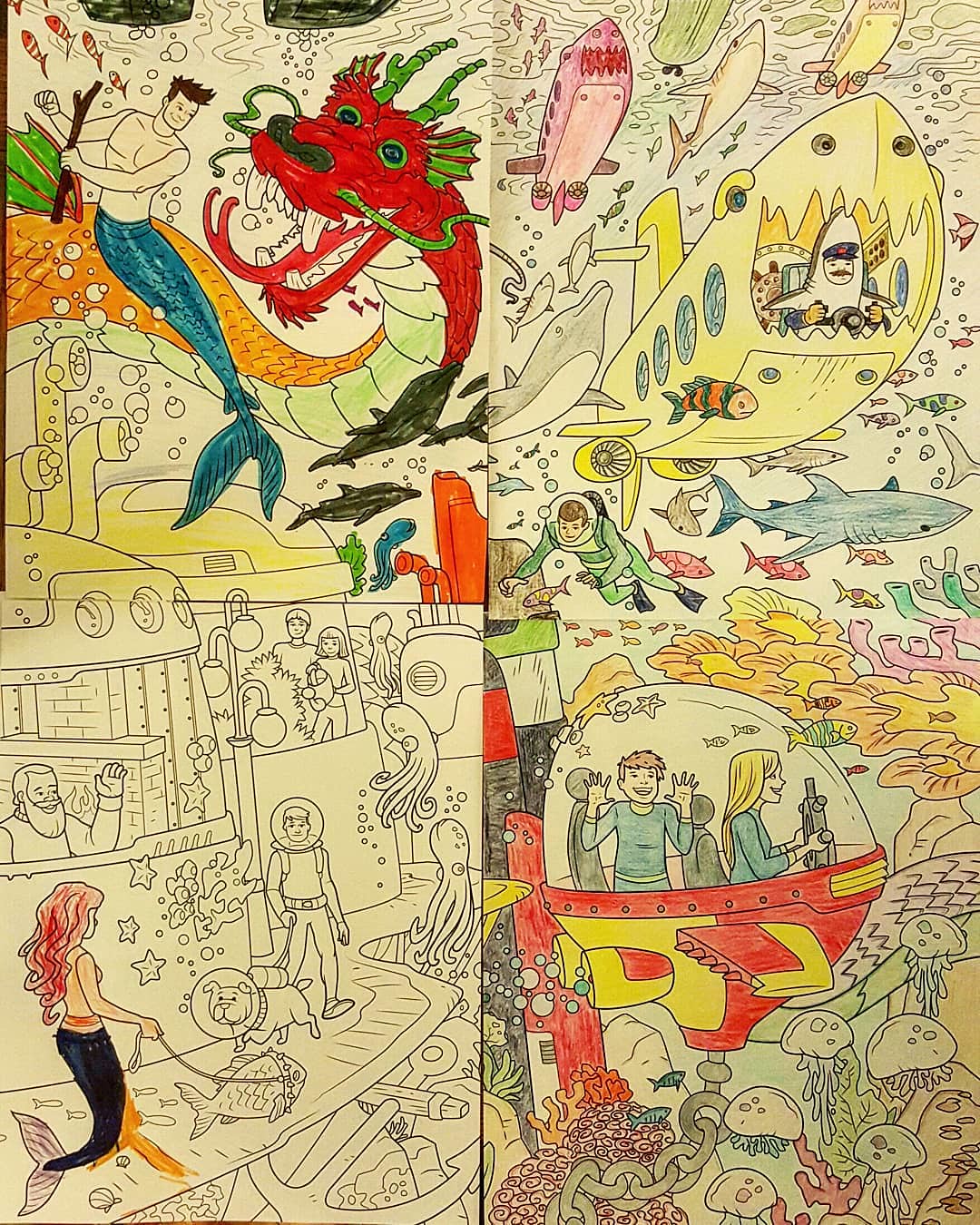The image consists of four partially colored illustrations from a coloring book, arranged in a two-by-two grid to form a larger scene. The top left quadrant features a bustling underwater city, possibly Atlantis, where a merman is depicted battling a Chinese dragon with a stick, while dolphins swim by. The top right section shows an array of shark-shaped submersibles, real sharks, dolphins, and other fish, as well as divers dressed in shark costumes. Below, on the left, a mermaid is seen walking a fish, juxtaposed with a man in a futuristic undersea suit walking his dog, both of which are likewise adorned in underwater suits. The bottom right quadrant illustrates a couple in a small submersible, seemingly anchored and observing an array of sea life, including jellyfish. The illustrations are detailed with pen and ink, highlighted with colored pencils, and some areas remain uncolored, suggesting that the artwork is unfinished.